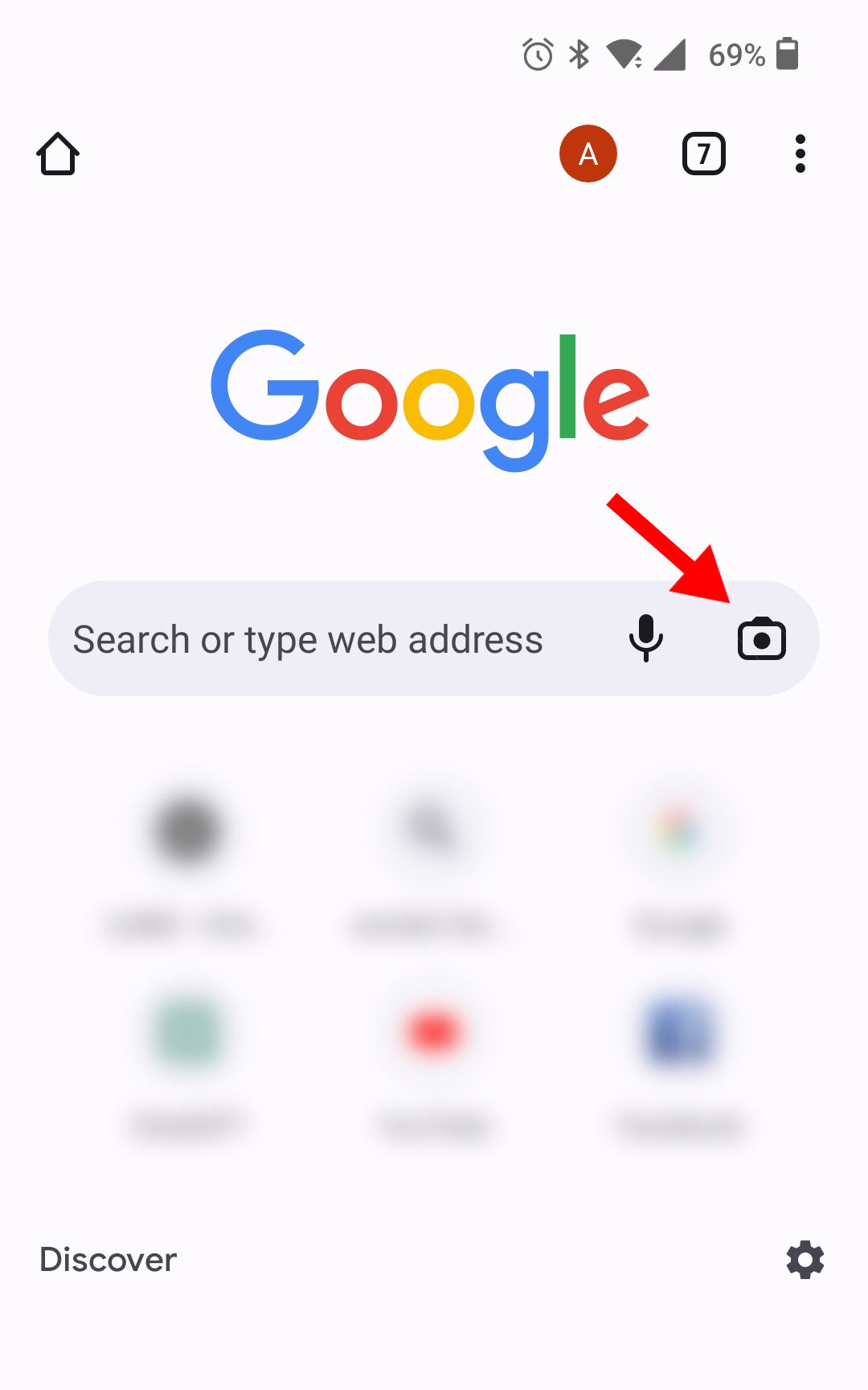On a pristine white background, the focus is on a digital interface displaying several icons and elements. Prominently visible is an alarm clock icon and a Bluetooth symbol. The battery indicator shows a 69% charge. There is an icon representing a house, a circle with a white letter 'A' inside, and a black square featuring the number seven. Three vertical dots are arranged in a line, which typically indicates a menu or additional options.

The layout features the Google logo in its classic colors: a blue 'G', followed by a red 'O', a yellow 'O', another blue 'G', a green 'L', and a red 'E'. A red arrow points to the camera icon located on the search bar, which also includes a microphone and camera icon to its right. The search bar itself has the prompt "Search or type web address".

Beneath the search bar, there are six small symbols, although they appear somewhat unclear or "blotched out." The fifth symbol is recognizable as the YouTube logo, and the sixth one is identifiable as the Facebook logo. At the bottom left corner of the interface, there is a 'Discover' section, while a settings icon is positioned on the right side.